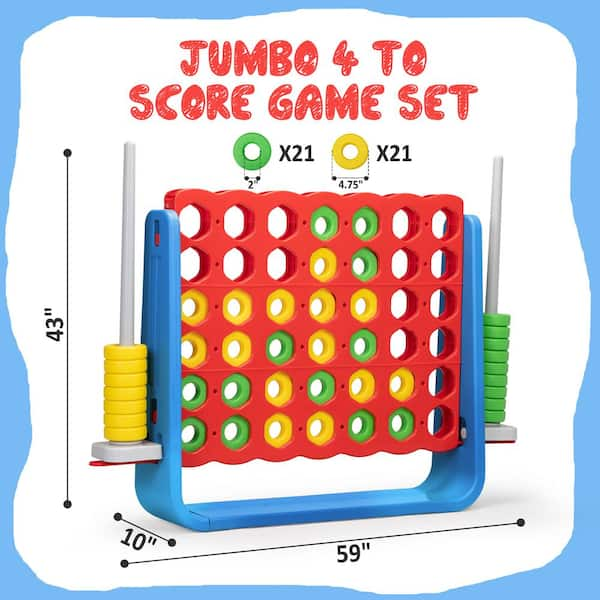This image is a product photo showcasing a large game set similar to Connect Four, named "Jumbo 4 to Score Game Set." The scene is set against a white backdrop with a wavy blue border that looks hand-painted. The game itself features a red grid with holes for dropping game pieces, held by a sturdy blue base. The apparatus is supported by gray poles on the left and right sides. The game pieces, green and yellow rings, are partially placed within the grid. The text on the top of the game reads "Jumbo 4 to Score Game Set" in scrawled red font. The dimensions, also displayed, indicate the game measures 43 inches tall, 10 inches deep, and 59 inches wide.